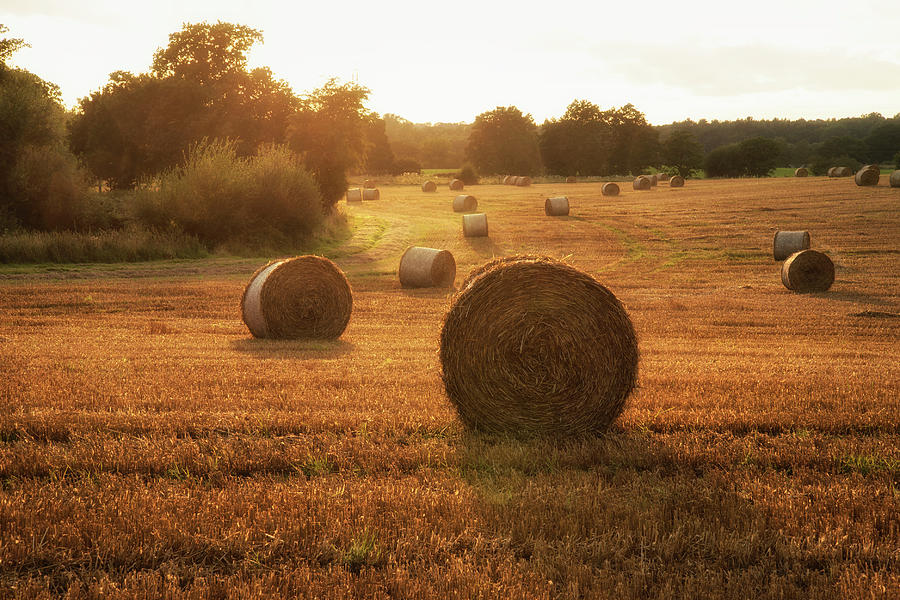The photograph captures a sprawling countryside farmland, bathed in the golden and orange hues of a setting sun. This warm, orangey glow suffuses the freshly mowed field, where large, cylindrical hay bales lay scattered across the landscape. Their number appears to be between 20 and 30, adding a rhythmic pattern to the bright yellowish-gold foreground, which gradually deepens into an orange-brown hue. The mowed lines in the field form a gentle arc around a grove of trees to the left, adding a dynamic flow to the scene. The tree line frames the field's edge to the right and wraps around the left side, suggesting the field's contour. The setting sun, low on the horizon and casting a brilliant white and gold light, enhances the serene and picturesque environment, with the entire forest visible in the distant background creating a tranquil countryside vista.